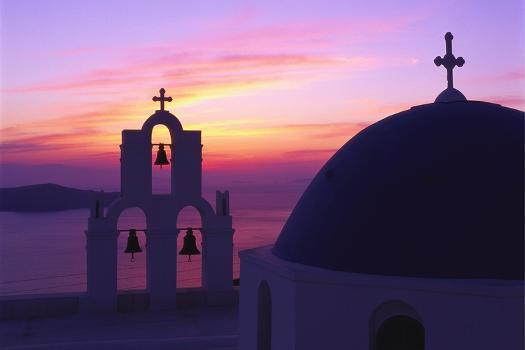This outdoor photograph captures a serene sunset over a coastal landscape, casting a mesmerizing blend of pink, orange, and purple hues across the sky and reflecting onto the ocean below. Dominating the right side of the image is a domed, white structure suggestive of an Orthodox or Christian church, topped with a cross. The dome descends into a larger, white base punctuated by windows, through which people could presumably access the roof. To the left of the dome, there is an open belfry with three silhouetted bells hanging inside cathedral-like arches, crowned by another cross. The bells and the church dome stand in silhouette against the vibrant, tranquil backdrop of the pink-tinted ocean and an island in the distance, highlighting the peaceful moment of sunset.